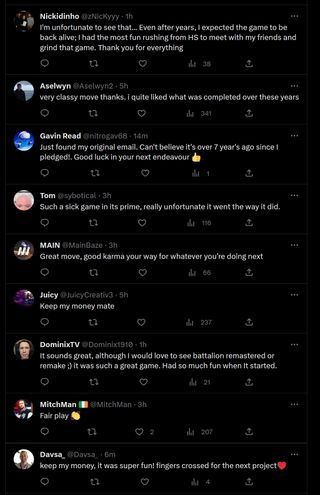**Caption:**

The vertical image depicts a series of nostalgic tweets lamenting the end of a beloved game. The background is black, with each tweet featuring the user's name, handle, and profile picture. 

1. **Nick (ID: ho@Nicky)**, one hour ago, expresses regret: "I'm unfortunate to see that... Even after years, I expected the game to be back alive. I had the most fun rushing from high school to meet with my friends and grind that game. Thank you for everything." Interaction options like retweet, comment, and like are visible.

2. **Aslyn (@Aslyn)**, five hours ago, appreciates the developers: "Very classy move. Thanks. I quite liked what was completed over these years. I think that's a great thing, kind of icons." Aslyn continues to reminisce about the journey, mentioning Gavin who found their original email after seven years and wishes good luck for future endeavors.

3. **Tom**, shares his sentiment: "Such a sick game in its prime, really unfortunate it went the way it did."

4. **Maine**, extends good wishes: "Great move. Good karma your way for whatever you're doing next."

5. **Juicy**, bluntly comments: "Keep my money mate."

6. **Dominic's TV**, expresses a desire for a remake: "It sounds great, although I would love to see Battlin remastered or remade. It was such a great game, had to post when it started."

7. **Mitchman**, gives kudos: "Fair play," with a clapping icon.

8. **Dobbs**, adds final thoughts: "Keep my money, it was super fun. Fingers crossed for the next project."

Each tweet combines personal memories and appreciation for the game while looking forward to future projects.